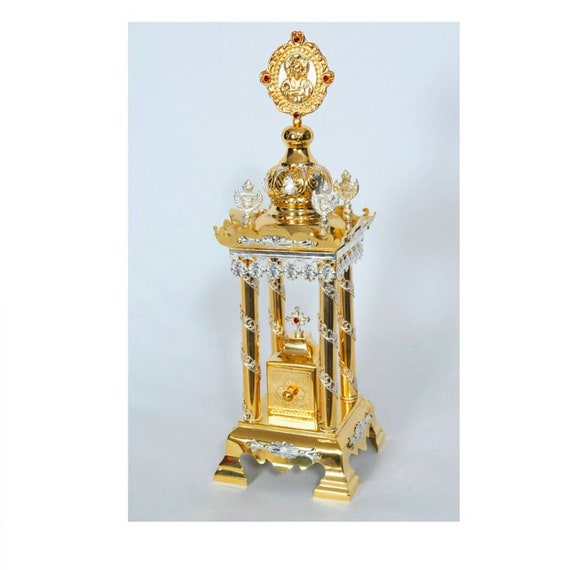This photograph captures an ornate, golden decorative item that closely resembles a miniature shrine or Catholic tabernacle. At its base, it stands on four short legs, supporting a cuboid-shaped platform that features a small drawer, likely intended to contain the Holy Eucharist. The central focus is a Christian cross, intricately mounted above this compartment.

Four cylindrical, spiraling pillars, adorned with diamond-like gems, ascend from the base to support a decorative roof. This roof is crowned with a tower-like structure which displays a circular medallion featuring an image of Our Lady holding baby Jesus, surrounded by three ruby-colored gems. Dazzling crystalline objects dangle from the perimeter of this top platform, adding to its intricate, trophy-like appearance. Glass angels grace the corners of the upper platform, enhancing the item's spiritual and gaudy aesthetic. The background of the image is a light gray, which highlights the golden, possibly brass, material of this elaborate shrine-like item.